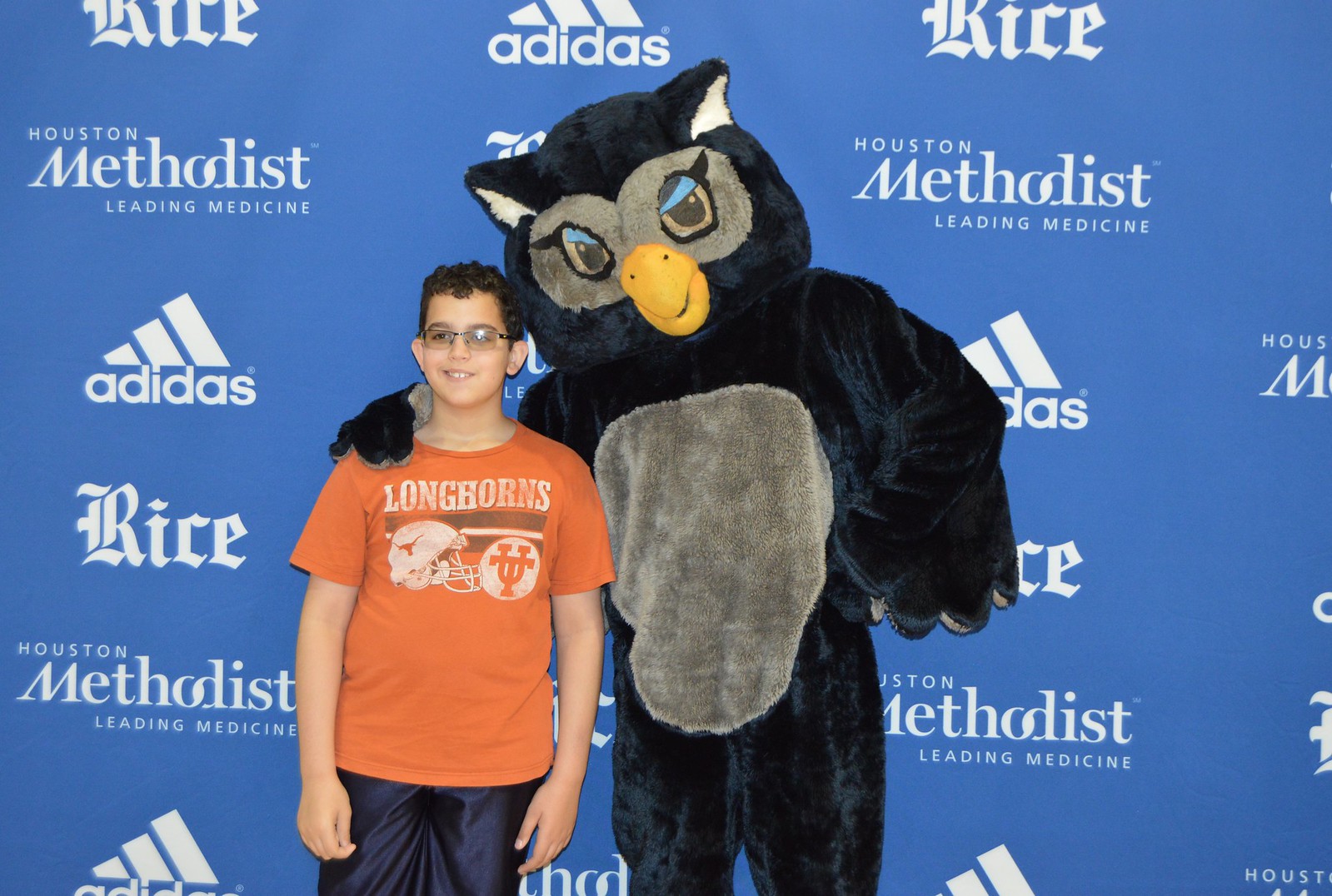A vibrant photograph captures a heartwarming moment between a young boy and Sammy the Owl, the beloved mascot of Rice University in Houston, Texas. The boy, who appears to be around 12 to 14 years old, has a light brown complexion and is sporting curly short black hair along with glasses. He is dressed in an orange T-shirt emblazoned with the University of Texas Longhorns logo and a football helmet, adding a touch of irony given the friendly rivalry between UT and Rice. The boy is smiling joyfully as Sammy the Owl, clad in a predominantly black costume with striking yellow eyes, a yellow beak, and distinctive blue and black lashes, wraps a comforting wing around his shoulder. Sammy’s costume features large gray circles around the eyes and white accents on the inside of the ears, adding to its detailed design. The background showcases a blue wall adorned with alternating logos of Houston Methodist Leading Medicine, Rice, and Adidas, enhancing the image's university and athletic theme. This delightful snapshot beautifully captures the spirit of camaraderie and school pride, blending elements of sportsmanship and community in a single frame.